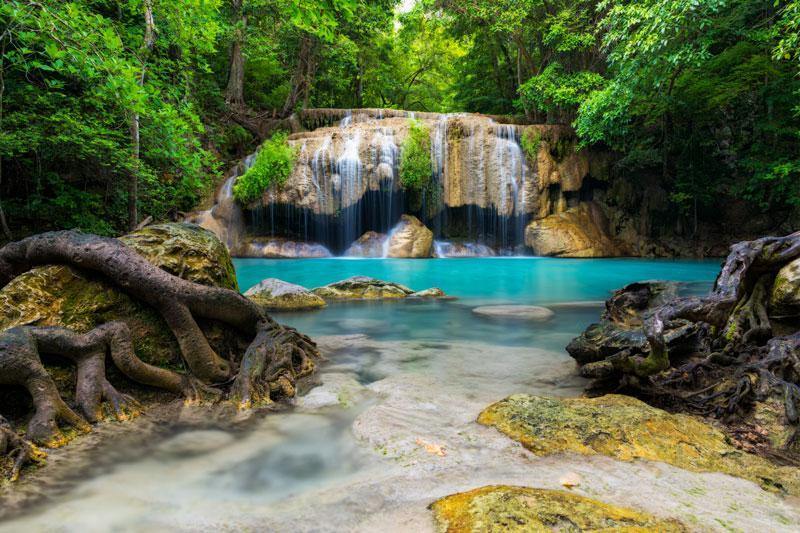This photograph captures a serene outdoor scene in a tropical forest. Centered in the image is a small waterfall cascading over a rocky ledge, which is adorned with moss and green foliage. The water tumbles just a few feet down into a bright aqua-blue pool that transitions to completely clear water toward the foreground. Flanking the pool, tree trunks or large roots snake over the rocks on both the left and right sides. In the background, just above the waterfall, a lush forest of trees with vibrant green leaves can be seen, likely growing on the sides of a river that feeds the waterfall. The colors in the scene range from golden yellows and light greens to forest greens and various shades of blue and brown, giving the entire setting a vivid, natural beauty. The stones framing the pool appear dark with hints of yellow, adding to the rich tapestry of the tableau. This picturesque spot is devoid of any visible wildlife or human interference, enhancing its untouched, tranquil atmosphere.